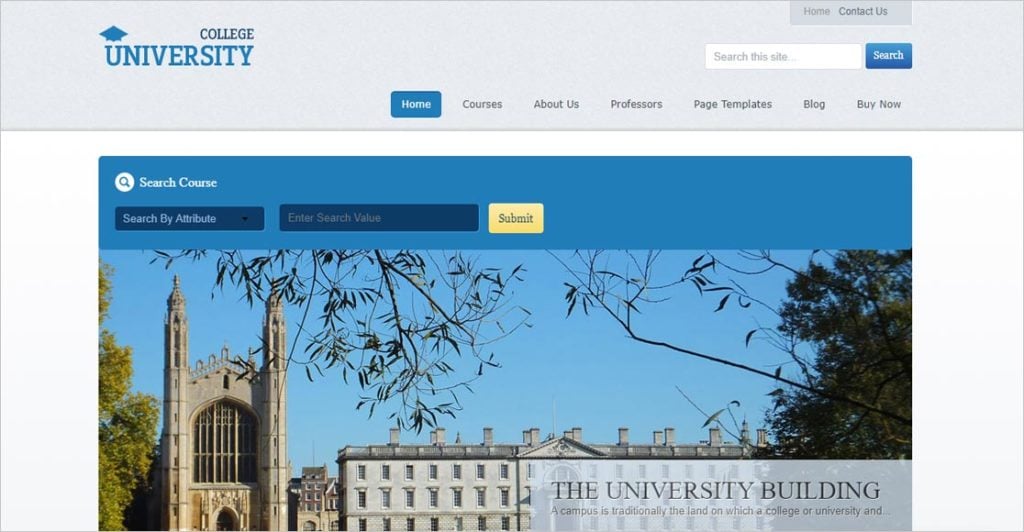The image is a screenshot from the website of College University. At the top of the page, there is a horizontal light gray navigation bar. In the upper left corner, the words "College University" are prominently displayed in blue, with a graduation cap symbol cleverly integrated over the "U" in "University." On the right side of this bar, there are links labeled "Home" and "Contact Us," followed by a search bar with a blue search button, where the word "Search" appears in white text.

Beneath this top navigation bar, centered at the top of the page, are several tabs labeled "Home," "Courses," "About Us," "Professors," "Page Templates," "Blog," and "Buy Now." Just below these tabs, the main image showcases a picturesque view of the university campus. The scene includes a blue sky, some verdant green trees, and a large building with a brownish-gray facade.

Superimposed on the bottom portion of the image, there is a section labeled "Search Course," accompanied by a search box and a submit button. In the lower right corner of the image, there is an informational section titled "The University Building," which contains additional details possibly about the building or the university itself.